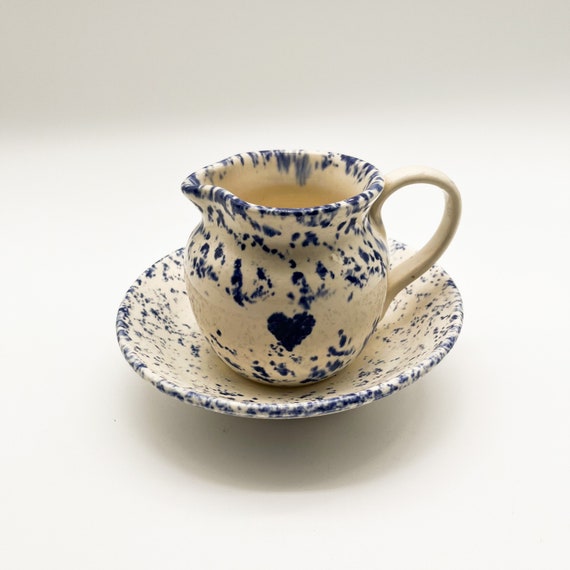The image features a ceramic cream pourer with a handle, delicately positioned on a speckled ceramic saucer. Both items share a cohesive design with an off-white base adorned with dark blue speckling. The pourer, ideal for serving milk or creamer, sports a spouted tip for easy pouring and a solid white handle. A notable feature is a navy blue heart in the center of the pourer, adding a distinct decorative touch. The accompanying saucer, more curved than flat but lacking the pronounced edges of a bowl, mirrors the pourer's speckled pattern and serves as a harmonious platform. The composition is set against a flat, white background, emphasizing the elegant simplicity and intricate detailing of the ceramic pieces.